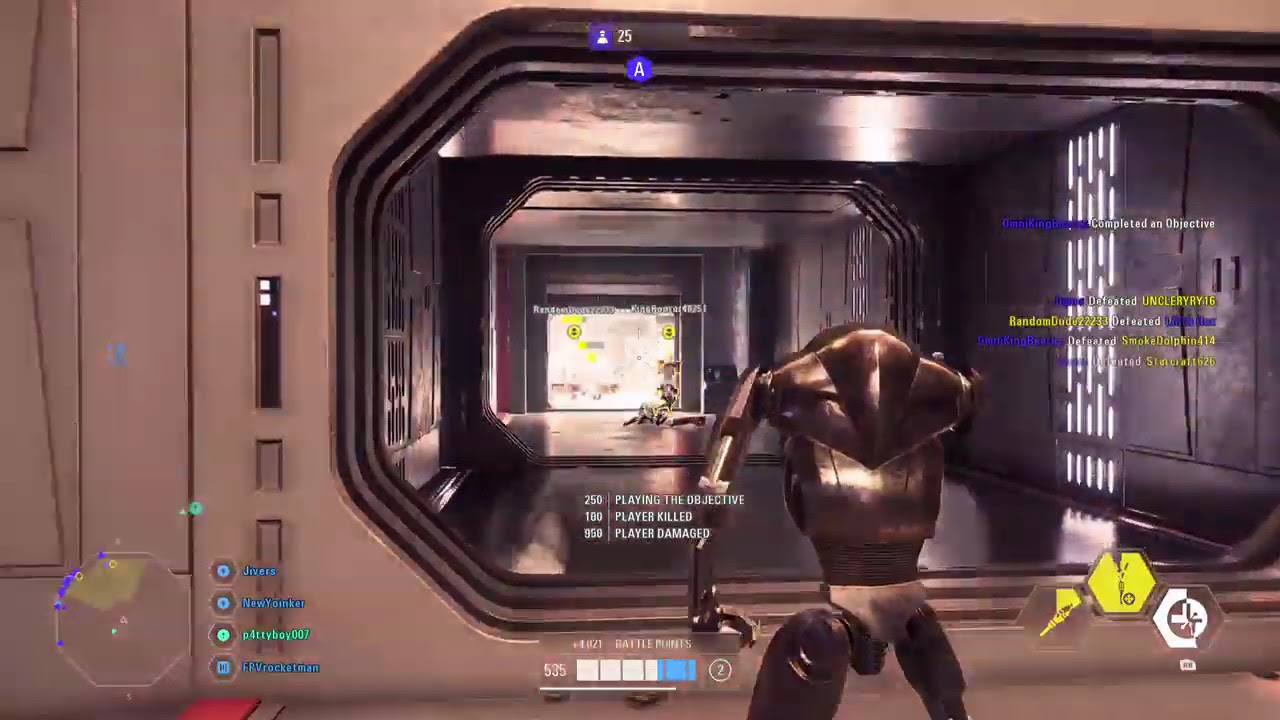The image depicts a scene from a futuristic video game set within a metallic-walled facility, possibly a starship or a high-tech factory. Central to the image is a bronze, humanoid robot with a blocky torso and no distinct head, only a low mound where a head would typically be. The robot stands in front of a tunnel-like opening with black framing, facing into the tunnel. Its right arm and both legs are visible, with the legs showing some variation in size that suggests a more complex design. Behind the robot, the environment is entirely metallic, composed of silver walls and floors. To the right of the tunnel, a whiteboard features yellow and brown parts. There are HUD elements scattered across the screen: a mini-map in the bottom left, gameplay icons in the bottom right, and various notifications and gamer tags indicating actions like "complete objective," "player killed," and "player damaged." The overall aesthetic is a mix of gray, white, yellow, blue, black, green, and red, and the image possesses a certain photorealistic quality despite its digital origins.